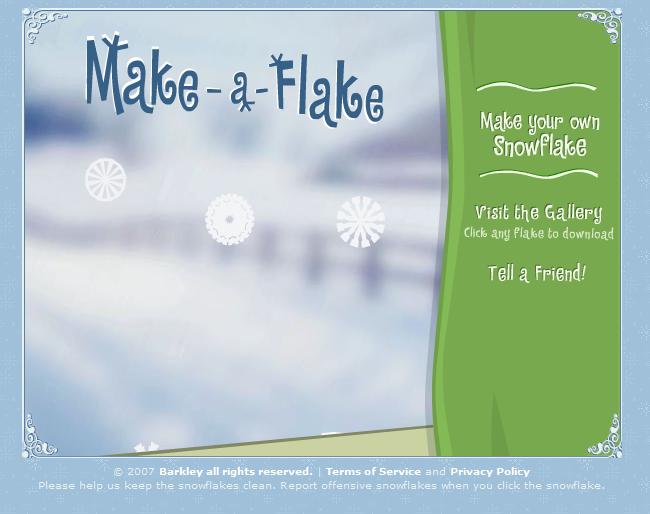The image, rectangular in shape and slightly wider than it is tall, is framed by a powder blue border with a pinstripe white line and filigree designs in the corners, creating a festive, Christmassy decoration. The image is entitled “Make a Flake,” with the title written in blue text at the top left. Below the title, there are three illustrations of snowflakes to click on. On the right side, a green background features the yellow text: "Make Your Own Snowflake, Visit the Gallery, Click Any Flake to Download, Tell a Friend." Below this, white print reads, "2007 Berkeley All Rights Reserve, Terms of Service and Privacy Policy. Please help us keep the snowflakes clean. Report offensive snowflakes when you click the snowflake." Overall, the inner part of the image is transparent or blurred, giving it a mysterious feel, while the footer and outer border provide a clean, organized frame.